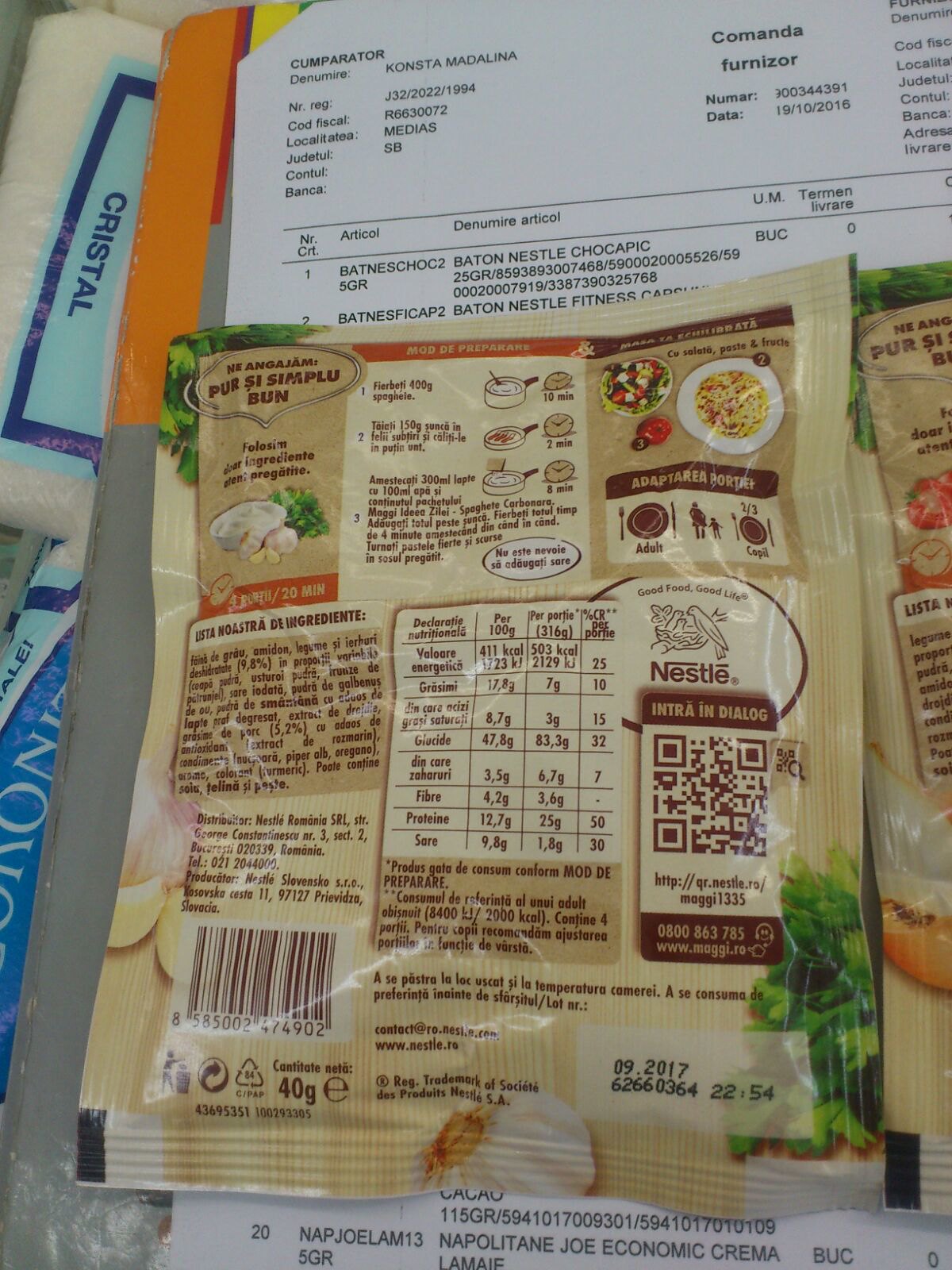The image portrays a variety of food items and packaging, centered around the purchase of steamed buns and other groceries. In the foreground, there is the backside of a plastic bag labeled "Percy's Simply Bun" at the top left, featuring an image of steam buns. The bottom right of the bag shows a printed date "09-2017" followed by the numbers "6266, 0364," and "2254." Additionally, the text on the packaging includes an ingredient list, nutrition label, and cooking instructions in another language, with illustrations indicating steaming methods and various dishes, including servings with vegetables, a tomato, and rice. There is also a section that appears to provide serving size information, marked with figures, a plate, and a reference to "two-thirds."

In the background, a receipt written in a different language spans across the image, featuring numbers and text. To the far left side, a bag of rice with a blue square labeled "Cristal" can be seen, suggesting additional contents within the plastic bag. Surrounding this packaging are illustrations of onions, garlic, and what seems to be conger eels. There is also a hint of a Nestlé product mentioned, contributing to the array of items possibly bought during this purchase. This detailed image serves as a snapshot of a diverse grocery haul centered around the steamed buns and other culinary essentials.